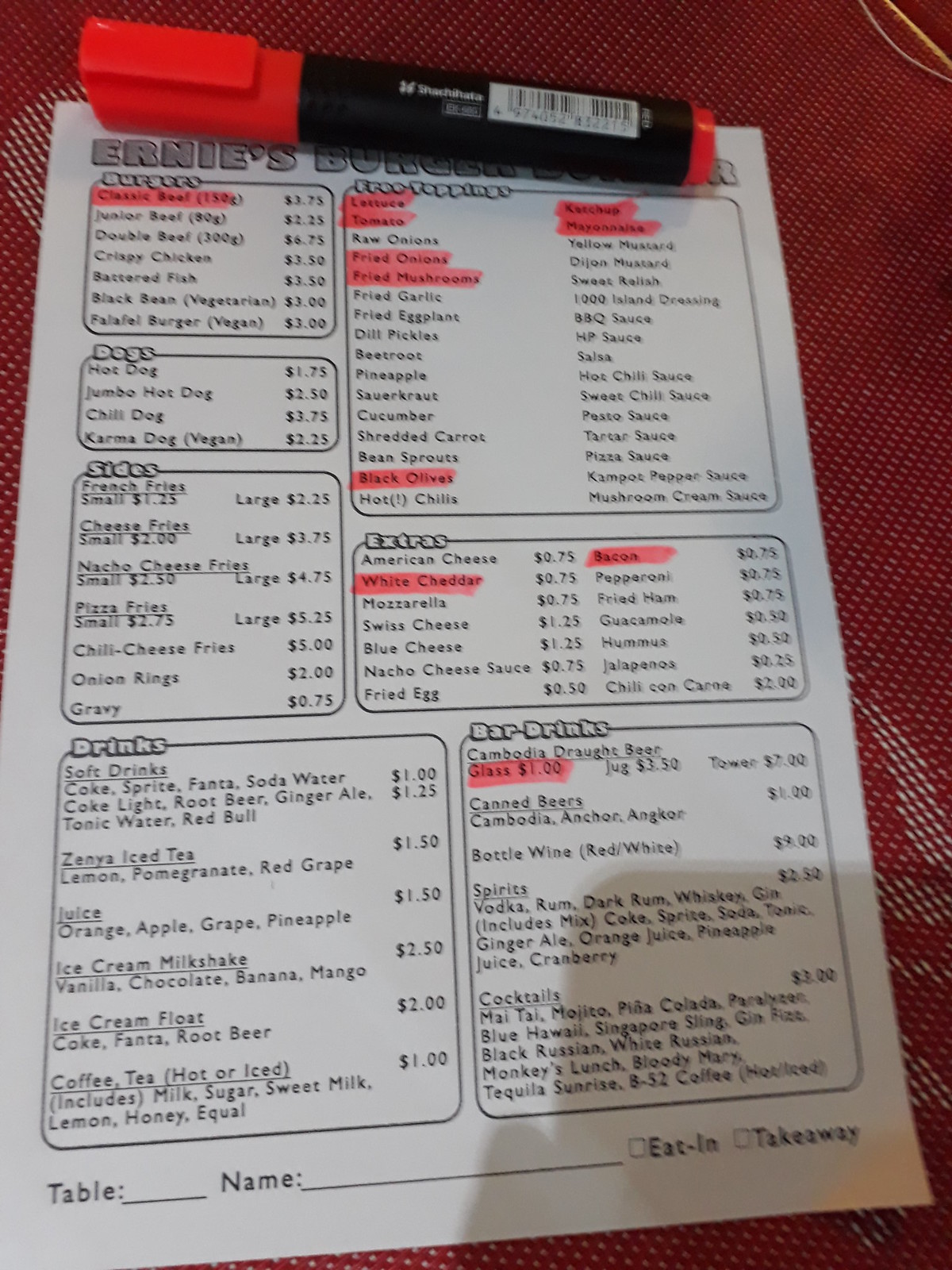This image depicts a photo of a menu set against a small, red, and white checkered plastic tablecloth. The menu itself is printed on plain white paper. At the top of the menu paper lies a red marker, partially obscuring some of the text. The visible section of the menu reads "Ernie's Burgers," although the marker conceals part of the lettering, making it difficult to fully discern.

Key items listed on the menu include a classic beef burger priced at $3.75, with a section for free toppings. The customer has marked their desired toppings, which include lettuce, tomato, fried onions, fried mushrooms, and mayonnaise. However, one of the highlighted items is unclear. In the extras section, they have selected additional options such as white cheddar cheese and tacos.

Toward the bottom of the menu, bar drinks are highlighted, featuring a glass of Cambodia’s draft beer for $1. This menu appears to be designed for customers to customize their orders by highlighting their preferred selections.